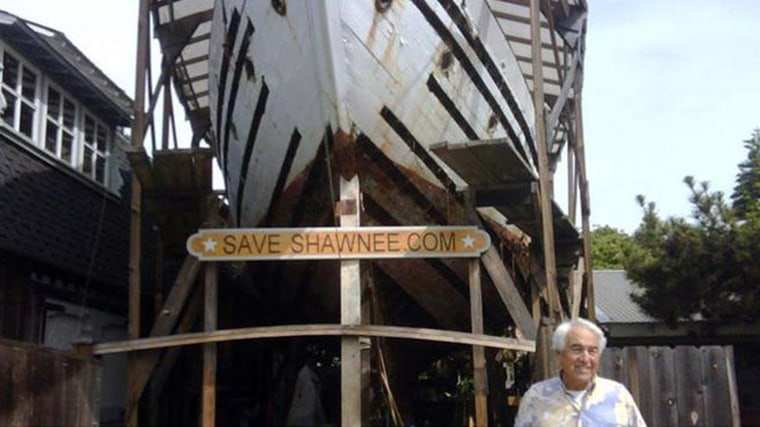This outdoor photograph, taken during the day under a clear blue sky, features a detailed scene centering on an old, white boat with black trim, which is perched on a brown wooden platform and secured with straps. The boat is prominently marked with a yellow sign that reads "SaveShawnee.com" in brown text, framed by two white stars. Below the boat, on the right side of the image, stands an elderly man with white hair, dressed in a white and blue multicolored shirt over a white t-shirt. He is smiling warmly at the camera. To the left of the platform, there is a large, two-storied building painted black or grey, with white-paned windows visible on the upper story. Adjacent to this building is another shed-like structure. The background is adorned with green trees, contributing to the picturesque, sun-lit environment. The overall scene leaves one pondering whether the sign is a campaign to save the vintage boat, with the man possibly being a supporter or caretaker of this preservation effort.